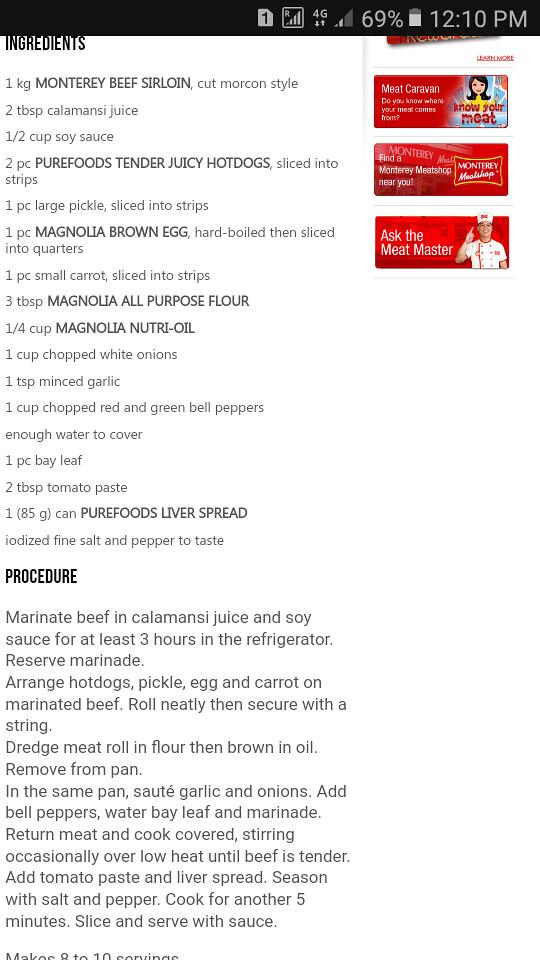The image appears to be a screenshot of a cell phone displaying a detailed recipe on a webpage. At the top of the screen, there is a black bar showing a battery icon at 69%, the time "12:10 PM", and additional icons in the center. Below the black bar, the word "Ingredients" is prominently displayed in large black letters. The ingredients list includes: one large Monterey beef sirloin cut Moroccan style, two teaspoons of calamansi juice, half a cup of soy sauce, two pieces of Pure Foods Tender Juicy hot dogs sliced into strips, one large pickle sliced into strips, one Magnolia brown egg hard-boiled and quartered, one small carrot sliced into strips, three teaspoons of Magnolia all-purpose flour, a quarter cup of Magnolia Nutri Oil, one cup of chopped white onions, one teaspoon of minced garlic, and one cup of chopped red and green bell peppers. It also specifies enough water to cover, one piece of bay leaf or one tablespoon of tomato paste, one package of Pure Foods liver spread, and salt and pepper to taste.

Adjacent to the ingredients, the word "Procedure" in capitalized black letters outlines the steps: marinate the beef in calamansi juice and soy sauce for at least three hours in the refrigerator and reserve the marinade. Arrange hot dogs, pickle, egg, and carrot on the marinated beef, roll it neatly, and secure with a string. Dredge the meat in flour and brown it in oil, then remove from the pan. In the same pan, sauté garlic and onions, add bell peppers, water, bay leaf, and the reserved marinade. Return the meat and cook covered, stirring occasionally over low heat until the beef is tender. Add the tomato paste and liver spread, season with salt and pepper, and cook for another five minutes. Finally, slice and serve the dish with its sauce.

On the upper right corner under the black bar, there are three red rectangles featuring white text and images of a person, likely related adverts or additional content on the page. The text related to the recipe includes details such as measurements, ingredient types, and specific brand names like Magnolia and Pure Foods, all listed in varying font sizes, with larger fonts for the headings and smaller print for the detailed lists and instructions.